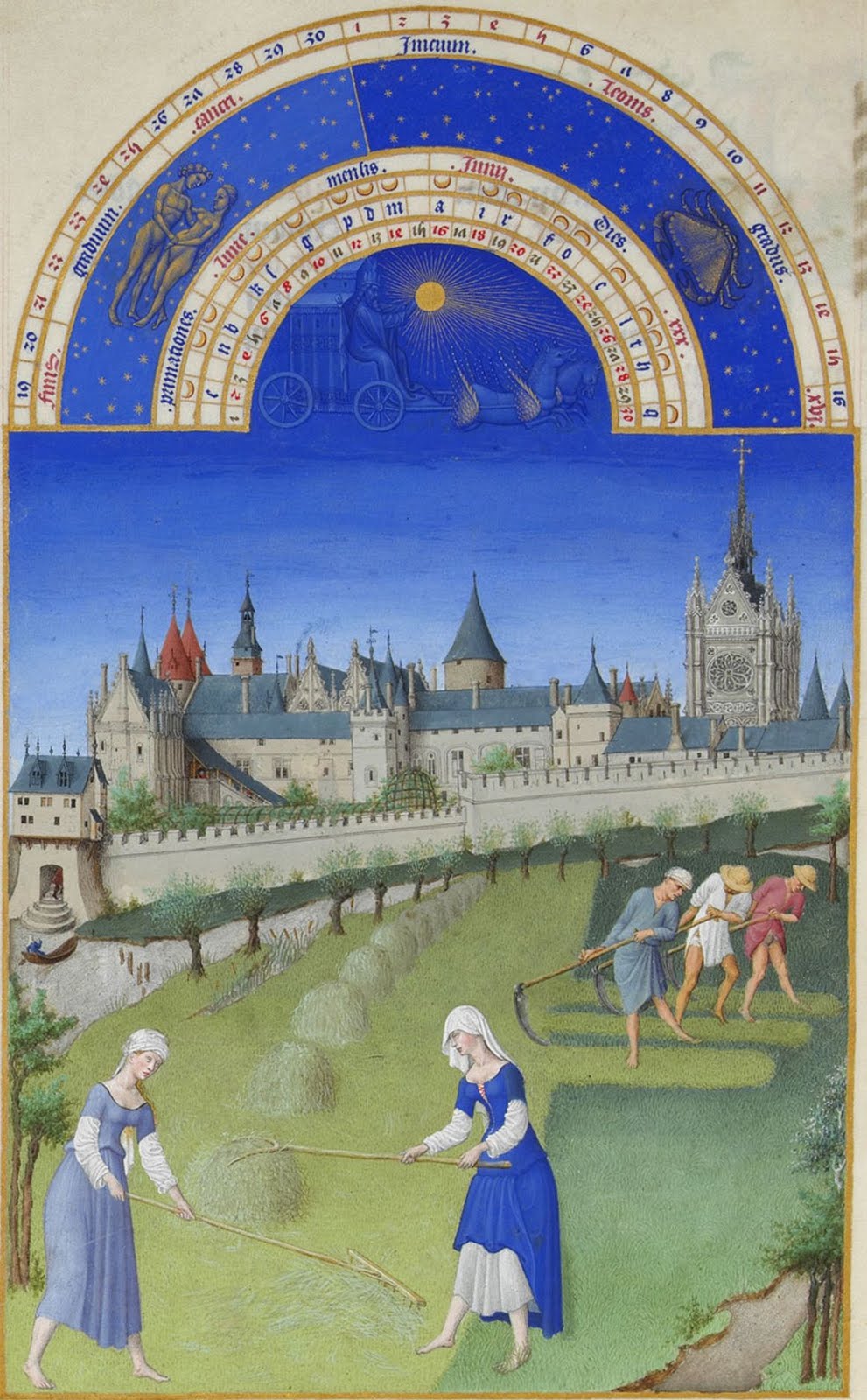This painting illustration portrays a vibrant medieval scene of peasants tending a field of crops in the shadow of a grand, grey castle with blue rooftops. The scene is filled with activity: in the foreground, two women are diligently raking hay, one dressed in a blue dress and bonnet and the other wearing a blue dress. Nearby, three individuals are seen wielding scythes, efficiently harvesting the green fields. The imposing castle, complete with turrets, a lookout tower, and a stone wall, dominates the backdrop, suggesting a historical setting. Above the pastoral labor, a peculiar dial with fantastical elements spans the top of the image. On this dial, a man holds up a bright, radiant light while driving a chariot led by two horses, one of which has wings. The dial also features enigmatic writing, moon symbols, and stars, with illustrations of a crab and a man and woman on its far ends. This elaborate composition captures the essence and daily life within a medieval landscape, blending the terrestrial toil of the peasants with celestial and symbolic imagery above.